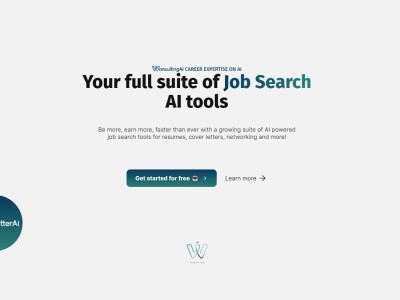The image showcases a sleek and professional webpage promoting a range of AI-powered tools designed to enhance the job search experience. Headlined "Your Full Suite of Job Search AI Tools," the webpage emphasizes benefits such as "Be More, Earn More, Faster Than Ever" with its growing array of tools for creating resumes, crafting cover letters, networking, and more. 

A prominent call-to-action button invites users to "Get Started for Free," encouraging immediate engagement, while a "Learn More" link provides additional details about the services offered. The branding prominently features the logo and brand name "Career Expertise on AI by WB Consulting." 

The design of the page is clean and minimalistic, maintaining a white background which adds to its simple yet professional aesthetic. The goal of the webpage is clear: to attract users to explore the AI tools for job searching through an enticing offer of a free trial, while also providing easy access to more in-depth information about the capabilities of the tools.